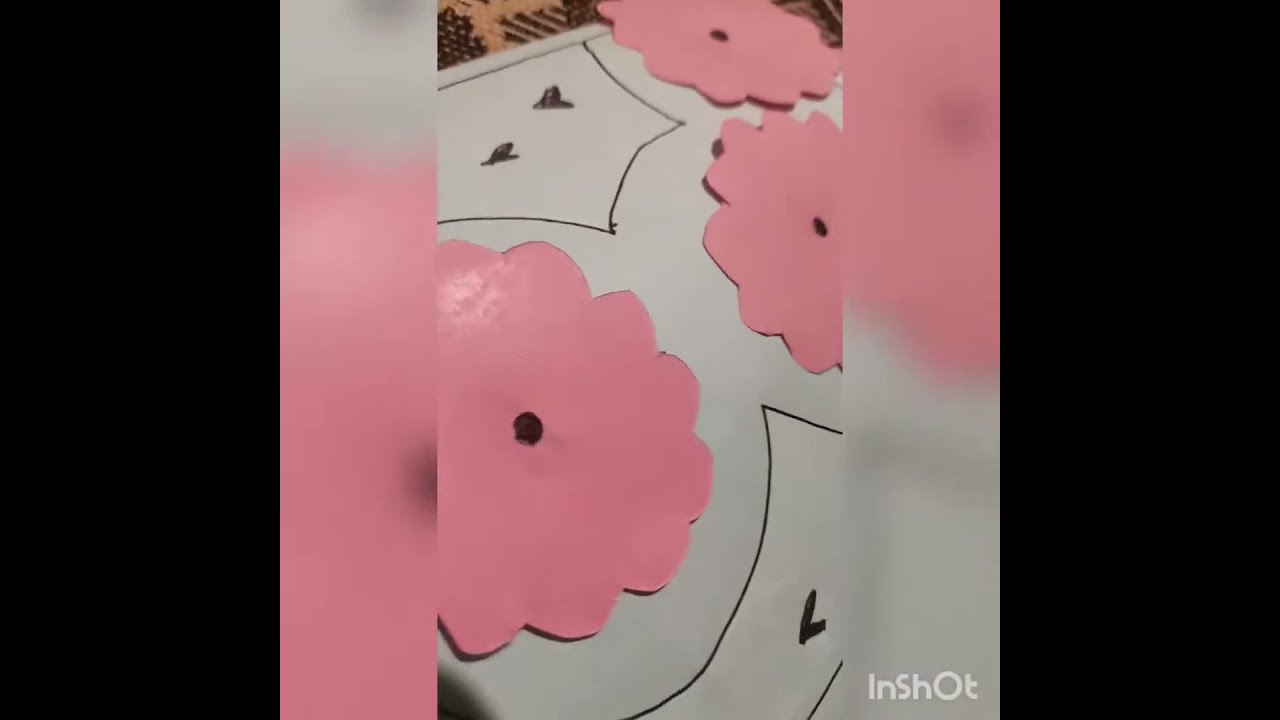The image features a muted bubble gum pink background adorned with an array of twinkling white shapes evocative of stars. These stars vary in size, with some appearing as small circles and others resembling plus signs or crosses with lines extending vertically and horizontally. In the bottom right corner, the word "InShot" is printed in a light white font, with a distinctive capitalization pattern: capital I, lowercase n, capital S, lowercase h, capital O, lowercase t. This simplified, starry scene includes approximately 12 to 15 starbursts, with a mix of smaller dots and larger glimmering stars. Thin black bars frame the image on the left and right sides, adding a structured border to the ethereal pink canvas.